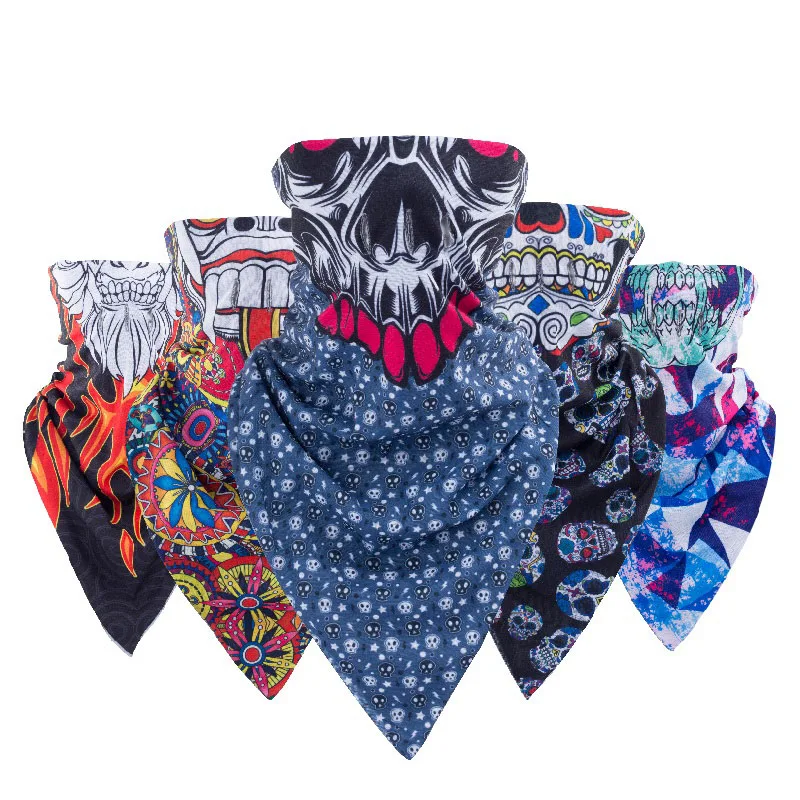This photograph features a series of five distinctive bandannas arranged against a stark white background, creating the illusion that they are floating in a white void. The bandannas are aligned in such a way that the leftmost and rightmost ones appear to be the farthest back, while those positioned center-left and center-right are slightly closer, with the central one being the most prominent. Each bandanna is topped with a unique skull design, leading into various themed cloth patterns below.

The center bandanna stands out with a stylized design displaying the bottom half of a skull, characterized by a large black nose hole and red teeth, suggesting it's missing its lower jaw, connected to a blue cloth adorned with white and black skulls. The leftmost bandanna features a bearded skull with sharp teeth, descending into a flame-patterned cloth. Next to it, the center-left bandanna has a Japanese demon Oni skull, complemented by vibrant Mayan patterning beneath it. The center-right bandanna showcases a white skull with long, sharp teeth, transitioning into geometric shapes of blues and pinks. The rightmost bandanna is adorned with a sugar skull design, leading into a black cloth with additional sugar skull motifs. The colors in the image span a spectrum from white, black, and gray to bright hues of yellow, orange, red, blue, pink, purple, and turquoise.

Overall, the image is meticulously composed, centering the bandannas and capturing their vivid details, making it suitable for product display, possibly for online retail platforms like Amazon.